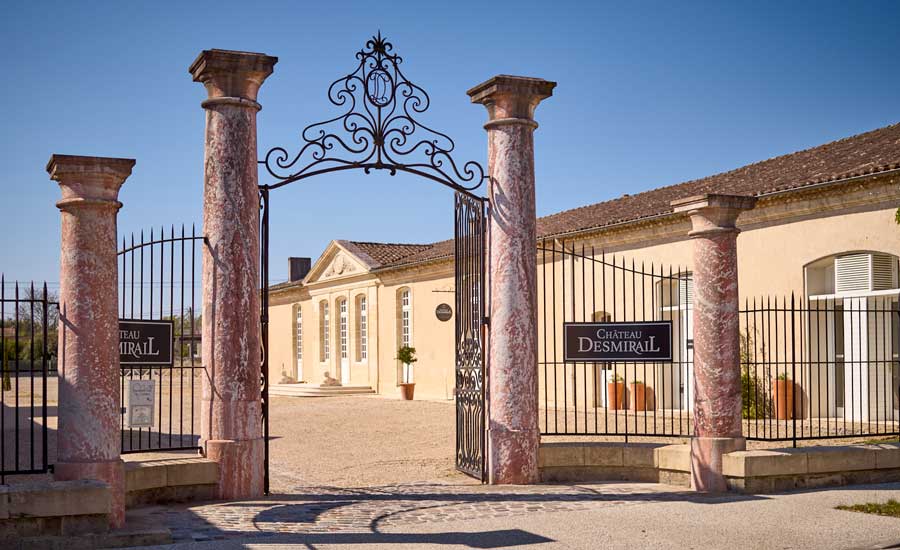The image depicts a grand tan building with a brown shingled roof, featuring tall arched windows. In front of the building stands a sophisticated black iron gate, which is currently open. The gate is adorned with an ornate, swirly decorative piece at the top that exudes a fairy-tale vibe, and incorporates an elegantly scripted letter 'D' within its design. This gate is flanked by four terracotta-like stone pillars, two large ones adjacent to the gate and two smaller ones further out, with additional black fencing connecting them. On either side of the entrance gate, black and white signs read "Chateau Desmerelles." The pathway leading up to the entrance is paved with stone, transitioning into brown gravel, and culminates in three steps that ascend to the doorway above which there is a slight peaked roof. The area within the gate appears to have some plants and space likely intended for parking, adding a functional aspect to the picturesque setting.